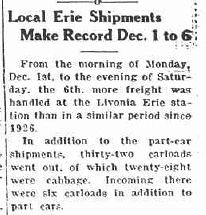The image is a black-and-white photocopy of a vintage newspaper column, slightly weathered and in an old serif font. The headline reads, "Local Erie Shipments Make Record December 1 to 6" in bold, upper and lowercase letters, and is followed by a centered underscore line. Below the headline, the text details that from the morning of Monday, December 1st to the evening of Saturday, December 6th, more freight was handled at the Livonia Erie Station than in any similar period since 1926. Specifically, 32 carloads, including 28 carloads of cabbage, were shipped out, while six carloads were received in addition to part cars. The square format and static-like imperfections near the top indicate it is a photocopy rather than the original clipping.